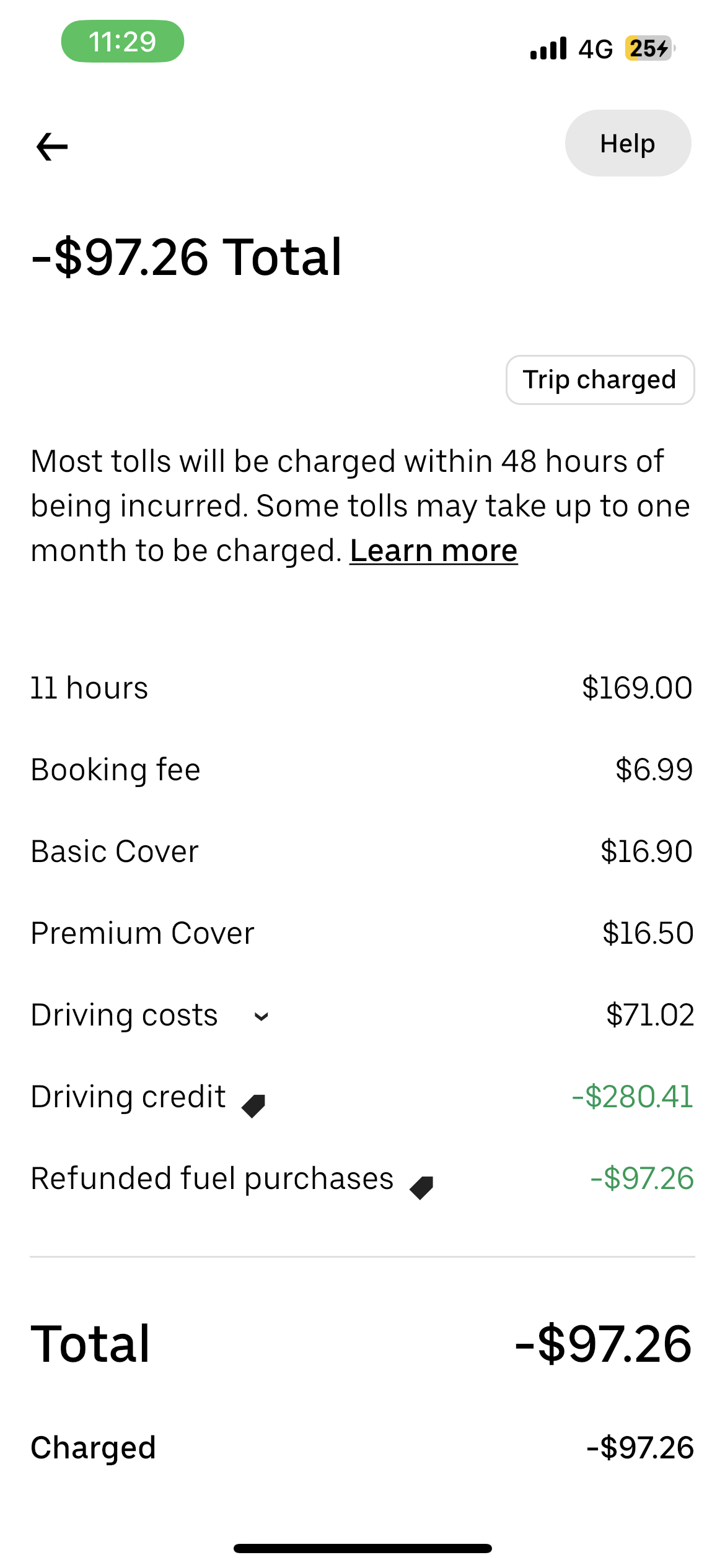The image depicts a screenshot of a toll account summary, though the specific company is not identified. The top of the screen displays the number "1129" in white against a green background, with standard icons indicating WiFi, 4G connectivity, and a battery level at 25%. A help button is located in the top right corner, and an arrow is on the top left.

Below this header, the account shows a negative balance of -$97.26. To the right of this balance is a small button labeled "Trip Charged." Text underneath explains, "Most tolls will be charged within 48 hours of being incurred. Some tolls may take up to one month to be charged." An underlined "Learn More" indicates additional information is available.

Itemized charges and credits are listed as follows:
- Fees: 11 hours for $169
- Booking Fee: $6.99
- Basic Cover: $16.90
- Premium Cover: $16.50
- Driving Cost: $71.02
- Driving Credit: -$280.41 (in green)
- Refunded Fuel Purchases: -$97.26 (in green)

These amounts culminate in a total balance of -$97.26, as indicated multiple times at the bottom of the summary.